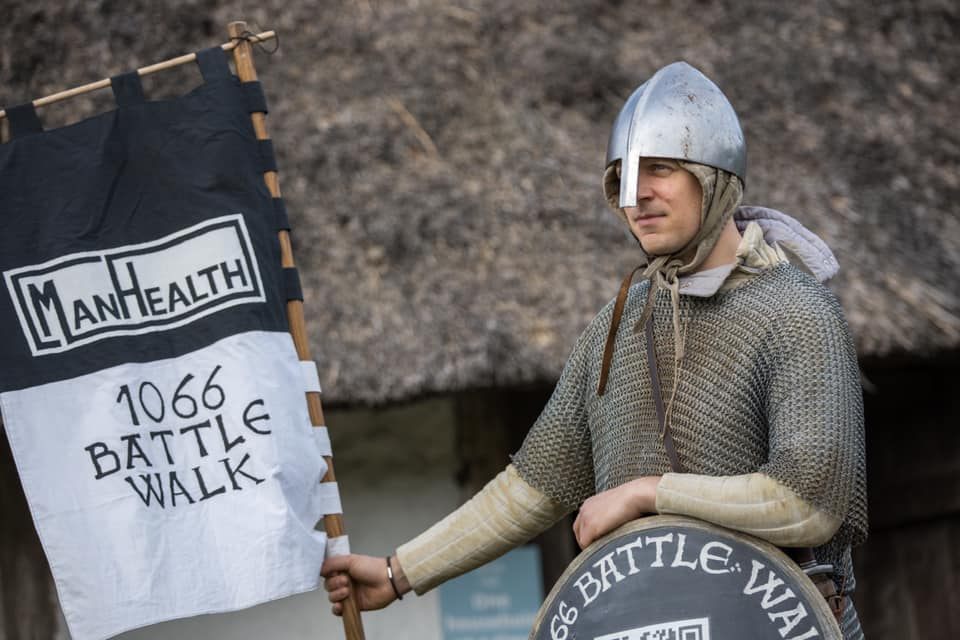This is a detailed photograph of a young man dressed in medieval battle armor, standing against a backdrop of a hut with a brown thatched roof. His outfit includes a silver helmet with a protruding nose protector, under which he wears a cloth head covering tied beneath his chin. He has layered garments: a gray chainmail over a beige-yellow undergarment, complemented by an old, possibly dirty, short-sleeve sweater over a long-sleeve one. In his left hand, he holds a flag that reads "Man Health 1066 Battle Walk," suggesting he is participating in a commemorative march. The piece of armor in front of him partially covers his mouth and one eye, leaving half of his face visible as he gazes into the distance.